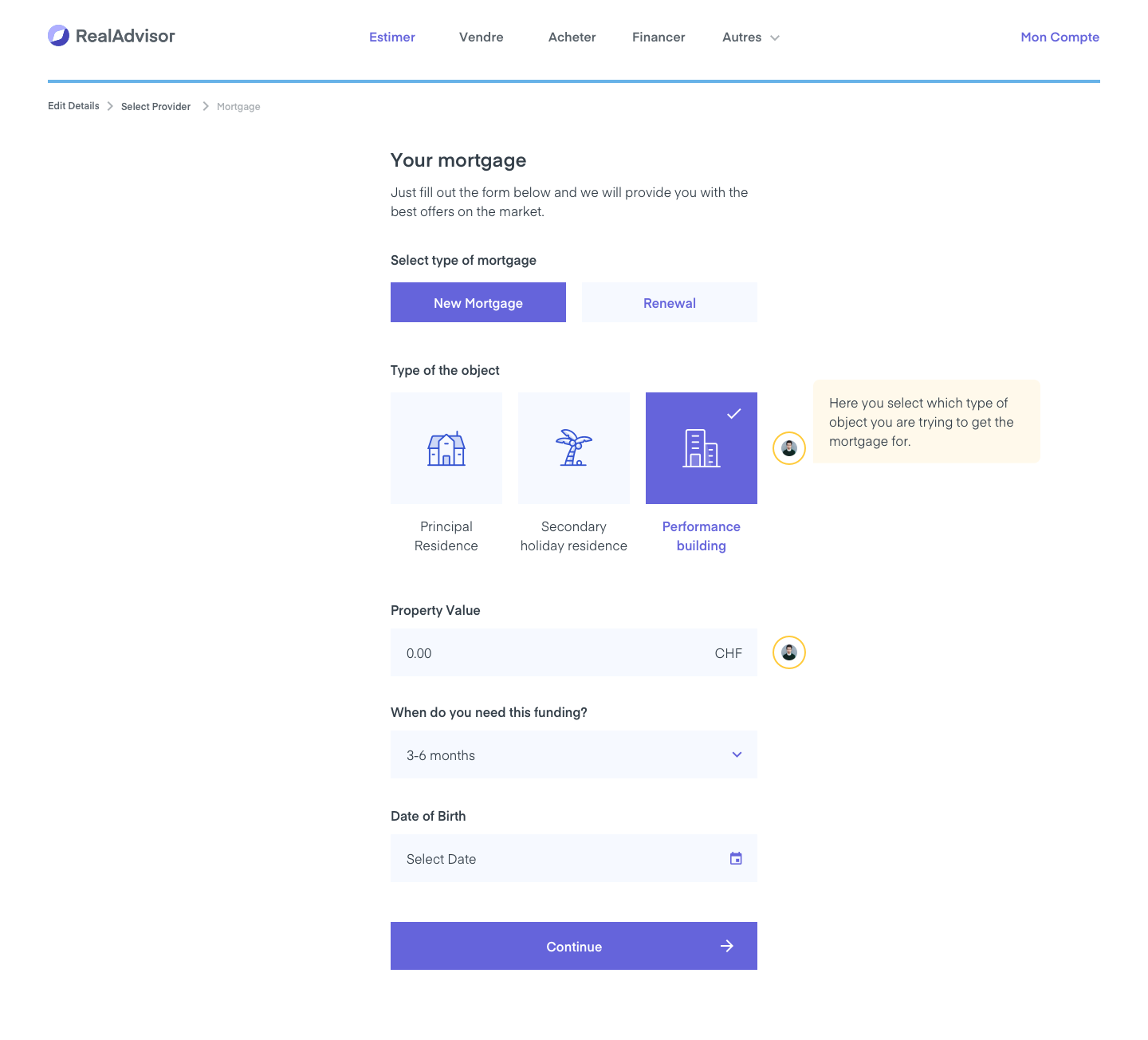The image displays a website interface for RealAdvisor, identifiable by its icon and name situated in the top left corner. The website's headings are primarily in French, with the 'Estimar' section currently selected. Beneath a fine blue line on the main screen, users can view and fill out details for mortgage inquiries. 

The first selection option allows users to choose between a new mortgage or the renewal of an existing mortgage, with 'new mortgage' highlighted in a purple button. The subsequent option is to specify the property type, with choices including principal residence, secondary holiday residence, and performance building; the latter is currently selected.

Users are then prompted to enter the property value, presently displayed as zero, to be input in Swiss francs or the applicable currency. Following that, there is a dropdown menu for selecting the required funding timeline, with 'three to six months' currently chosen. Additionally, there is a date selector for entering the user's date of birth. At the bottom of the screen, a purple 'continue' button is visible for progressing further in the form.